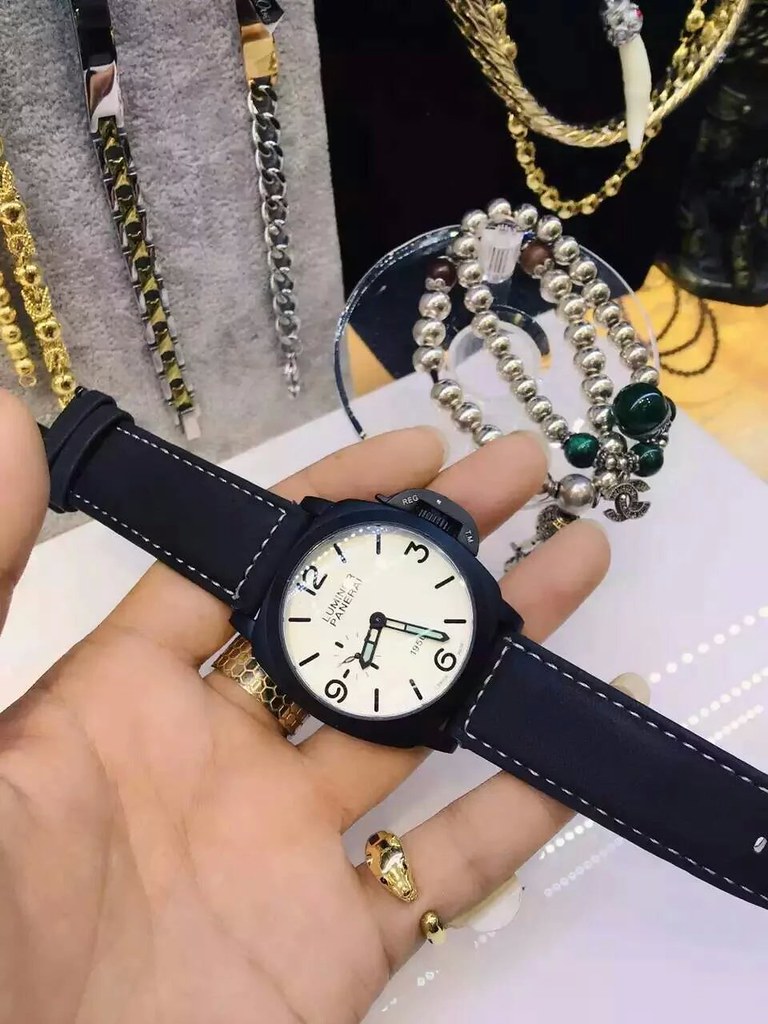The image showcases a close-up of a hand holding a black wristwatch, prominently positioned in the lower left corner. The hand is oriented palm-up, revealing the forefingers, thumb, and a gold ring adorning the middle and pinkie fingers. The wristwatch has a sleek, black leather strap and features a white face with distinct black numerals. The background reveals additional details: a white table stretches out beneath the hand, and in the upper left corner, a board displays four chains—two gold and two silver—partially visible. In the upper right corner, against a black backdrop, hang two more gold chains. Below these, resting on a white plate on the table, is a piece of jewelry, possibly a bracelet, crafted from silver with an arrangement of silver and green beads.